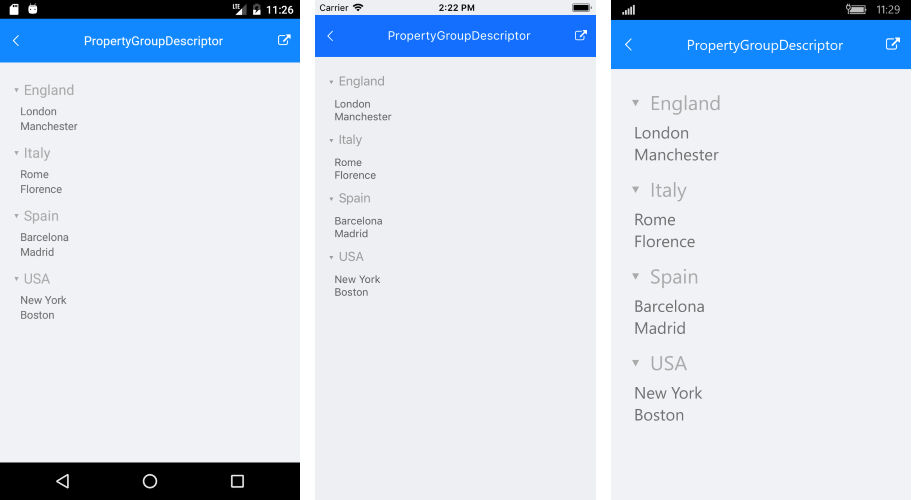The image displays a webpage with a white background and three distinct panels. 

**Panel 1:**
- The top of the panel features a black border, containing icons for a SIM card, a plug, and a battery indicator. The modem status shows "LTE" and a cell signal with the time "11:26."
- Below, a thick blue banner stretches across the panel, featuring a white left arrow icon and the text "Property Group Descriptor" in white, all combined into a single word.
- On the right side of the banner is a square icon with an arrow pointing upwards into the top right corner, reminiscent of the "2" or "1" positions on a clock face.
- The rest of the panel has a gray background populated with a list of locations: "England, London, Manchester, Italy, Rome, Florence, Spain, Barcelona, Madrid, USA, Newark, Boston."

**Panel 2:**
- The top section against the gray background shows the word "Carrier," a Wi-Fi signal icon, the time "2:22 PM," and a battery indicator.
- Following this, a blue banner similar to Panel 1 is present, with the text "Property Group Descriptor," a left arrow icon, and a square with an arrow pointing upwards.
- The list below remains unchanged, displaying the same locations: "England, London, Manchester, Italy, Rome, Florence, Spain, Barcelona, Madrid, USA, Newark, Boston."

**Panel 3:**
- The black top banner of this panel includes a cell signal indicator, the battery icon showing the time "11:29."
- The blue banner, repeating the style of the previous panels, houses the left arrow, the "Property Group Descriptor" text, and the square with the upward arrow icon.
- The gray background beneath it continues to display the list of locations: "England, London, Manchester, Italy, Rome, Florence, Spain, Barcelona, Madrid, USA, Newark, Boston."

Overall, the webpage's three panels maintain visual and textual consistency, with each panel reflecting network status icons, identical navigational banners, and the same set of global locations.